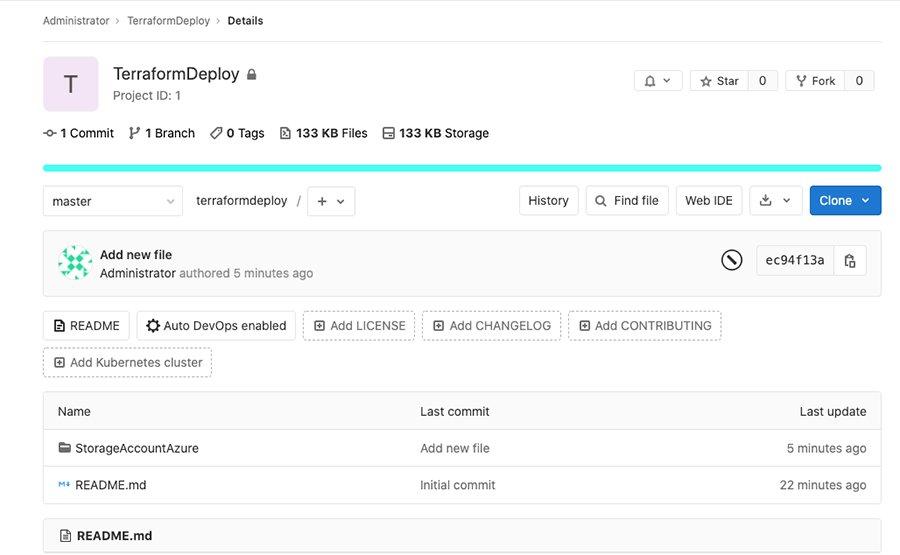The image depicts a user interface screen with a white background and various elements organized in a structured manner. At the top, gray lines provide structural division, and text labels read "Administrator," "Terraform Deploy," and "Details." Below this, a gray box with a "T" icon and the label "Terraform Deploy" is present, accompanied by a lock icon and the text "Project ID 1."

Additional details within the gray box include indicators for "1 comment," "1 branch," "0 tags," file size "133 KB," and storage usage "133 KB." Three buttons are aligned at the top, represented by a bell, a star, and a fork icon. A blue line divides this section from the one below.

Underneath, there's a box containing the labels "Master" and "Terraform Deploy," with plus and down-arrow icons adjacent to them. Action buttons labeled "History," "Find File," "Web IDE," "down-arrow," and "blue clone" are organized in a row.

A noticeable component is a blue box containing a green-circled icon and the text "Add New File," along with the status "Administrator Authorized 5 Minutes Ago." On the right side, features include a circle with a line through it, an "EC94F13A" button, and several labeled buttons: "Read Me," "Auto DevOps Enabled," "Add License," "Add Change Log," and "Add Kubernetes Cluster."

A light blue box follows, detailing columns such as "Name," "Last Commit," and "Last Update." Below this are elements like "storage account," "Azure," and an update note "Add New File 5 Minutes Ago." The entry "ReadMe.md" is marked with "Initial Comment 22 Minutes Ago." Finally, a blue box with a paper-like icon labelled "ReadMe.md" is evident, providing additional context.